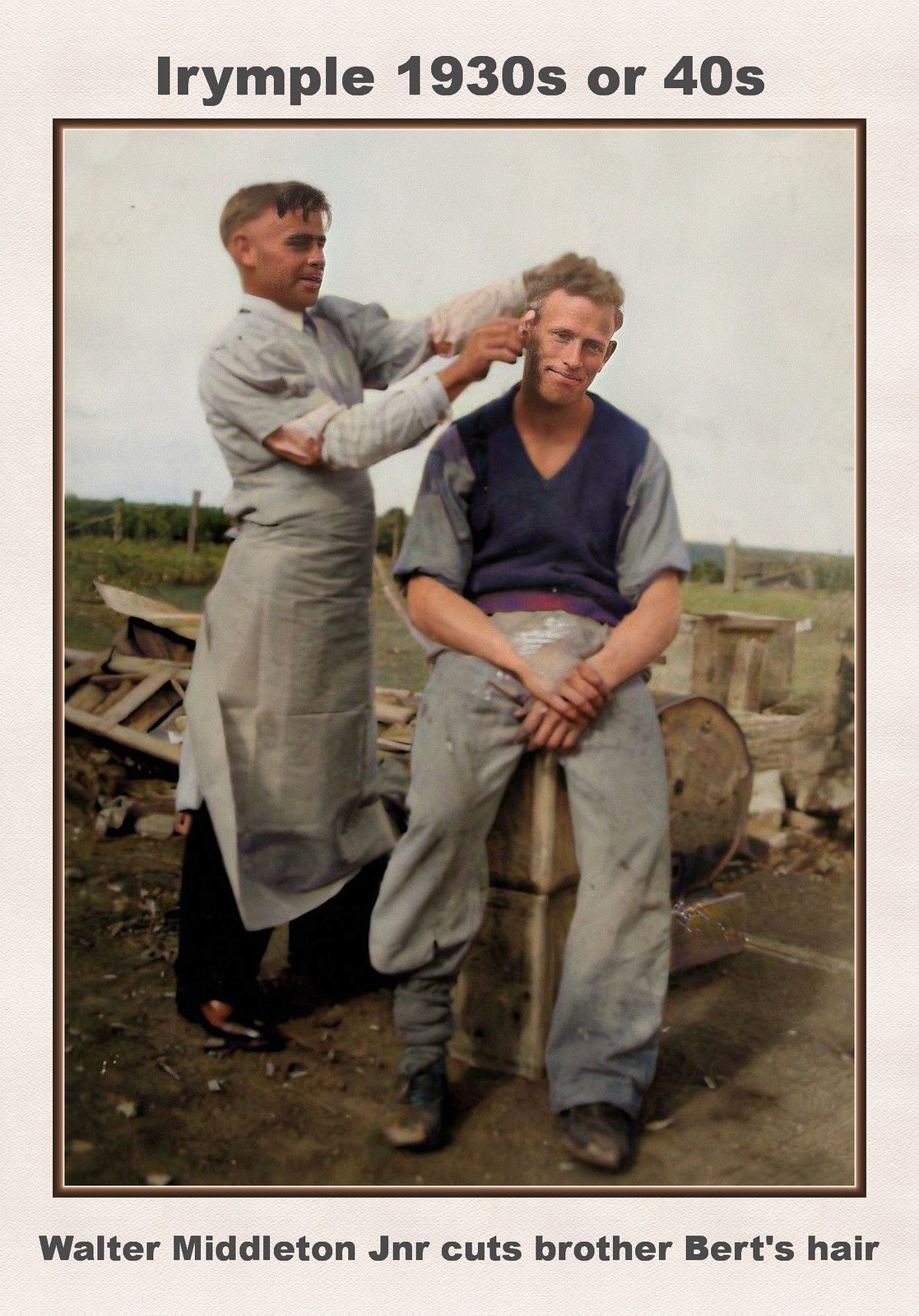This is an old photograph from the 1930s or 40s, possibly an advertisement. The image features two white men outdoors in a rural farm setting. The top of the photo has the text "I-R-Y-M-P-L-E, 1930s or 40s," while the bottom reads "Walter Middleton Jr. cuts Brother Burt's hair." Burt, who is getting his hair cut, is sitting on wooden farm equipment, possibly a box or barrel. He is dressed in a dark blue top with gray sleeves and gray pants, and he has a slight smile as he looks at the camera. Walter Middleton Jr., the man cutting Burt's hair, is positioned to the left and is wearing a white apron over black pants, a button-up shirt, and dress shoes. He is holding shears and working on the right side of Burt's head. The background features a large, open field under a gray sky, with various wooden objects, including a ladder and a barrel, scattered around. The image has a white border with a brown trim, adding to its old-timey feel.